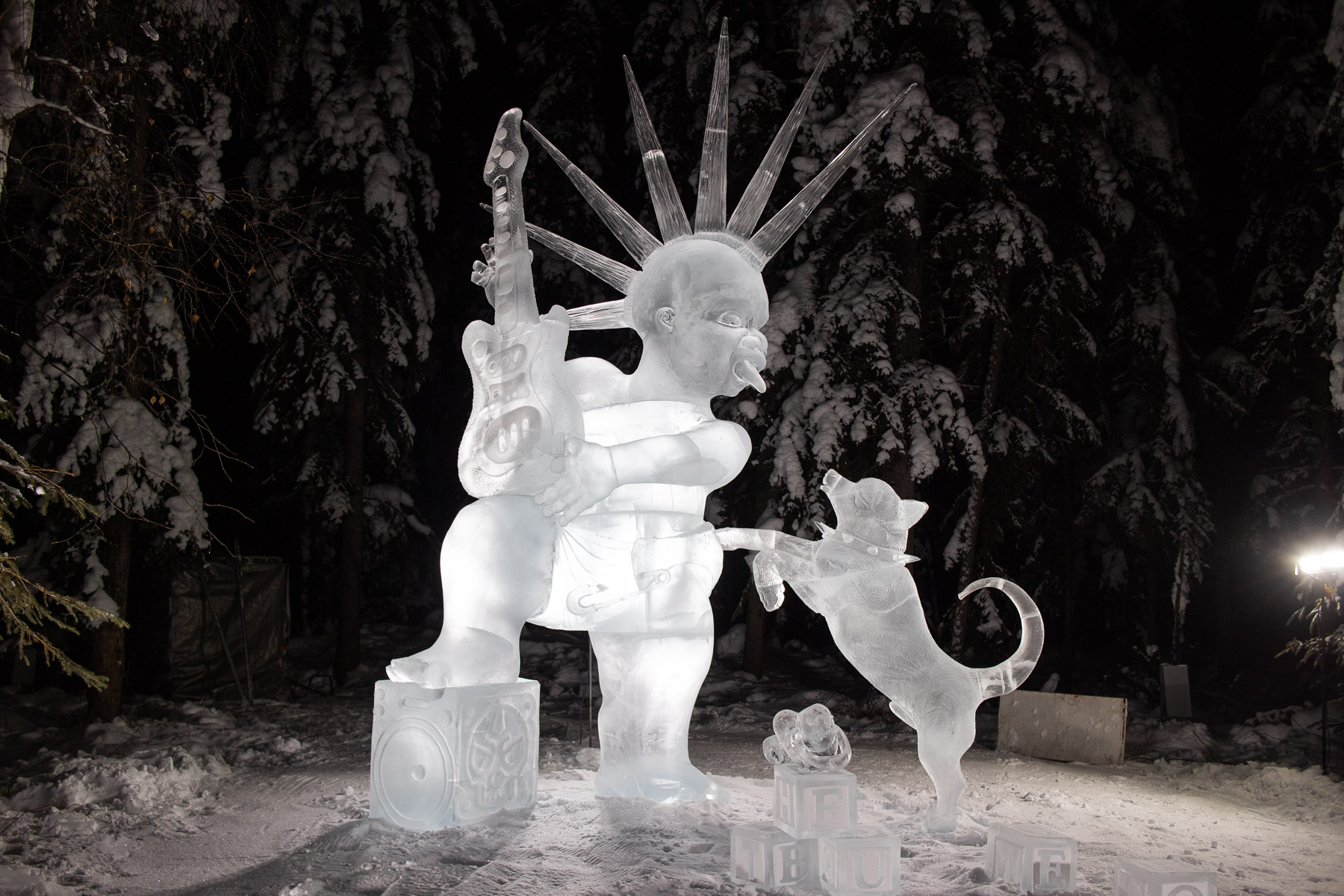The image depicts a detailed nighttime scene captured in black and white, emphasizing the subdued colors that enhance the wintry landscape. Snow blankets the ground, and the background showcases evergreen trees heavily laden with snow, their branches drooping gracefully towards the ground. Dominating the foreground is a meticulously crafted ice sculpture featuring a cherubic, slightly chubby young figure with a mischievous expression, characterized by spiky, ice-formed hair reminiscent of a punk rock style. This impish figure, possibly representing a toddler punk rocker, is poised with one knee resting on what seems to be an amplifier while holding an electric guitar. The positioning of the guitar is vivid, with one end of it cradled by the figure's left arm and the neck gripped by the right near shoulder height. The figure is playfully sticking its tongue out at a small ice-sculpted dog, likely a chihuahua, which stands on its hind legs, one paw pressed against the figure's side, gazing up with curiosity. In front of the figure, there are several ice-carved children's blocks with visible letters like B, U, F, and possibly E or F. The entire scene is dramatically illuminated by a spotlight positioned on the right side, casting a magical glow on the ice sculptures and making the intricate details of the figures and the snowy landscape come to life.